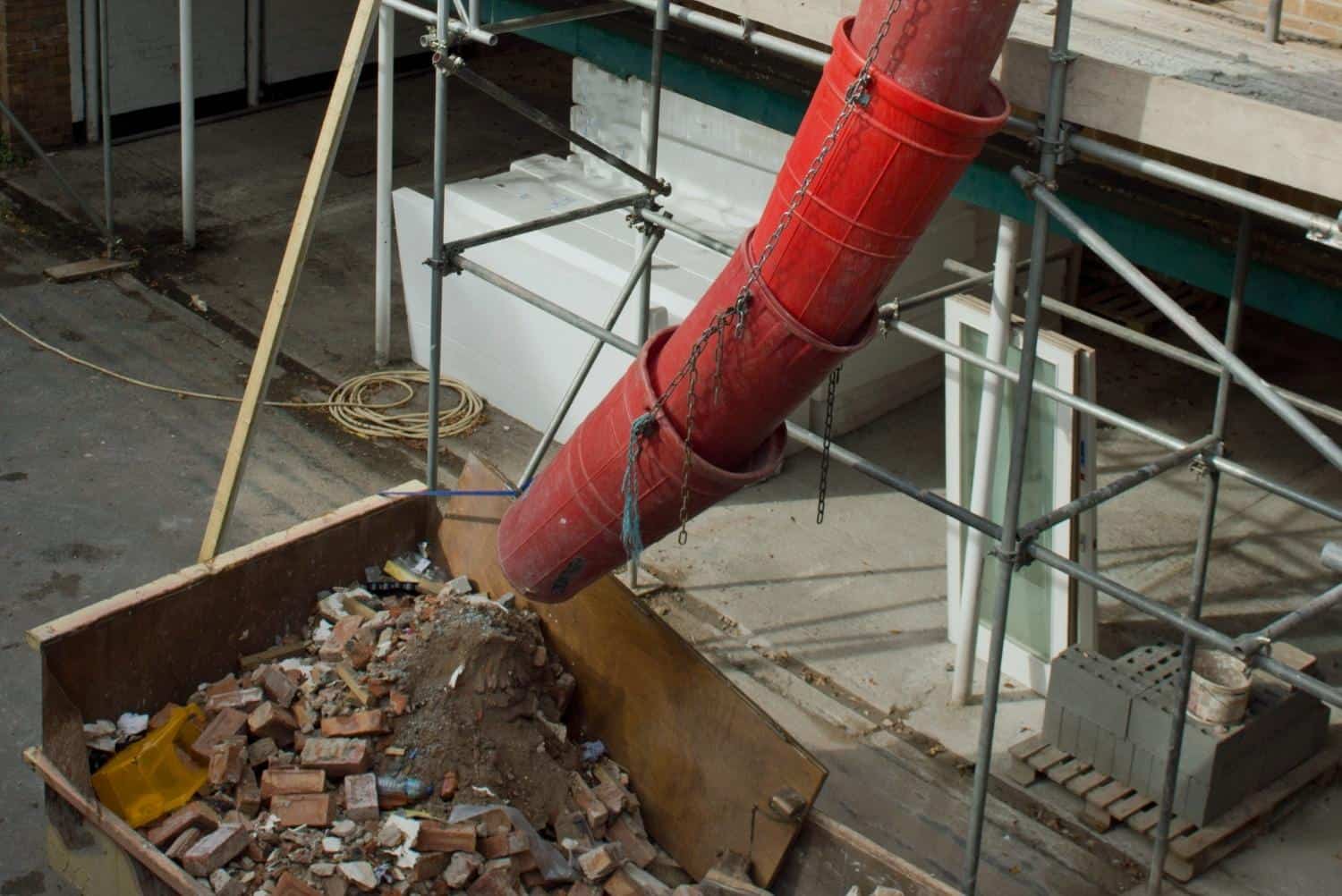The image depicts a bustling construction site viewed from an elevated angle. Dominating the scene is a long, segmented red tube assembled from multiple buckets and connected with metal chains, which channels debris from an upper level down into a large, rusted dumpster below. The dumpster is filled with a variety of demolition debris, including bricks, dirt, paper, and other waste materials. Surrounding this setup, the area is dominated by metal scaffolding and construction framing, with visible concrete flooring and steps in the background. Additional construction materials such as cement bricks, wood paneling, rope, and extension cords are also scattered around, contributing to the busy environment. In the background, parts of the building under construction or renovation can be seen, along with windows and other structural elements.